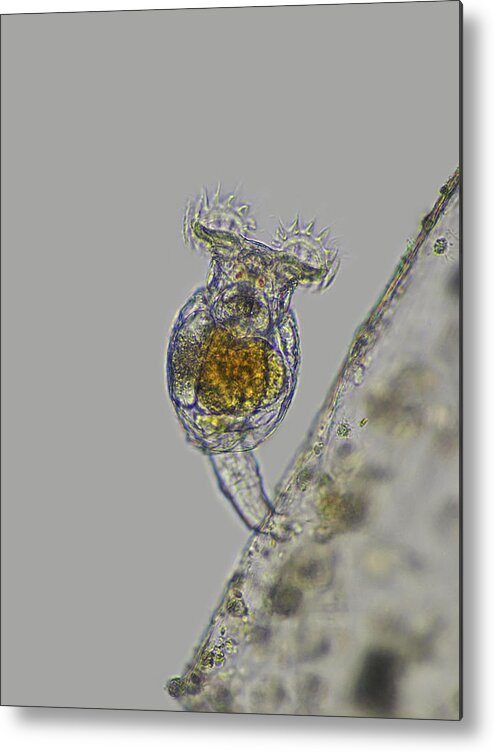The image under the microscope reveals a fascinating scene with a detailed gray background. Dominating the center, there is a clear, gelatinous organism with a round body and an oval-shaped head. The creature features two spiky protrusions that resemble budding flowers or horns and extend from its head. Positioned to the lower right side, a triangular gelatinous mass is partially visible, adorned with small, bubble-like structures that enhance its translucent appearance. The organism appears to be intricately connected to this triangular mass via a root-like tail. Suspended within the clear body of this enigmatic creature is a blob of orangish-yellow material, possibly indicative of a nucleus. Overall, the image, though ambiguous in origin or magnification, highlights a potentially single-celled or small multicellular organism in what could be a detailed microscopic study.